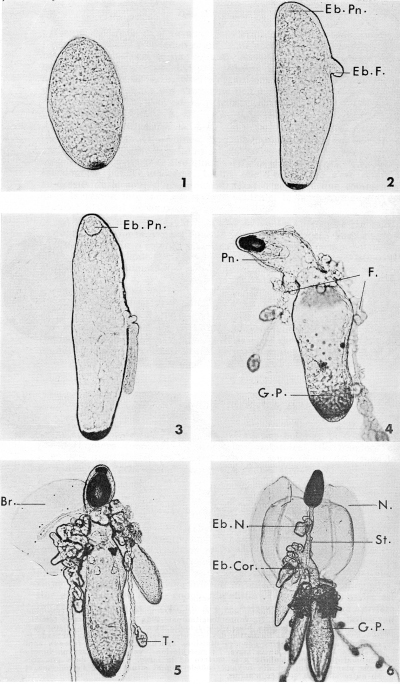The image consists of six black and white diagrams, each labeled from 1 to 6 in the bottom right corner, depicting the progressive stages of a biological structure, likely a microorganism. 

- **Frame 1:** A simple vertical oval with a small black spot.
- **Frame 2:** The oval elongates, has a lobe labeled "EBPN" at the top, a smaller lobe labeled "EBF" on the side, and a black dot at the bottom.
- **Frame 3:** The oval further elongates, with the black dot still present. A small rectangular shape drifts downward from the side, while a curved black area labeled "EBPN" appears at the top.
- **Frame 4:** The oval now shows a constriction near the top, which bends left, with a large black dot labeled "PN." Small ovals labeled "F" extend from the main body's sides, and a dark spot labeled "GP" is at the bottom.
- **Frame 5:** The oval has a large black dot on top and receives additional attachments on the left and right, including a drooping rectangle with black dots labeled "BR" and a small sac labeled "T" at the bottom right.
- **Frame 6:** Similar to Frame 1 but with added features: strings with black dots hang from the bottom, a long stalk labeled "ST" connects the black dot to the main oval body, a now-expanded circular area labeled "N," a twisted part labeled "EBCOR," a square object labeled "EBN" on the stalk, and the main oval labeled "GP."

Overall, the diagrams illustrate the transformation and increasing complexity of an oval structure through successive stages.